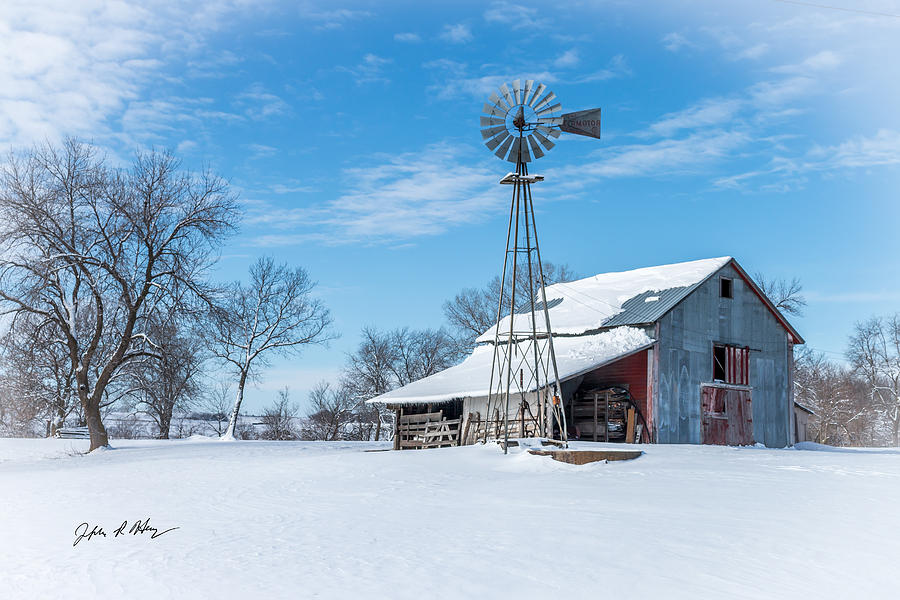This image showcases a large, rustic barn in the midst of winter. The barn is mainly gray due to weathered wood but has distinct red-painted interior sections visible through small openings. The roof is three-quarters covered in a thick layer of snow, with a metal sheath exposed on the top where the snow has melted slightly. Adjacent to the barn, an aged wooden fence stands, adding to the pastoral scene. In front of the barn, there’s a silver windmill, apparently in motion, and its slender form towers over the snowy landscape. To the left, several bare trees with branches capped with snow frame the scene, indicating the frigid, leafless season. The bright, blue sky overhead is filled with wispy, puffy clouds, allowing ample daylight to illuminate the snow-covered ground that completely surrounds the barn. The combination of these elements captures the serene, yet stark beauty of a winter day in the countryside.